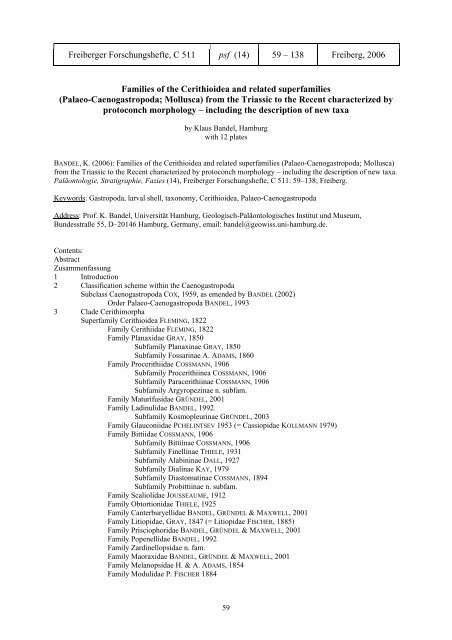The image depicts a simple black and white print piece on a white background with no border. At the top, there are four rectangular boxes with exceedingly small text. From left to right, the boxes read: "Frye Burger C511," "PF14," "59-138," and "Fryeburg 2006." Below these boxes, in darker black text, there is a title that states: "Families of the Cerithodea and Related Superfamilies from the Triassic to the Recent, Characterized by Proto-conch Morphology, Including the Description of New Taxa." The entry notes the contribution of Klaus Bardell from Hamburg and mentions the inclusion of 12 plates. Though the rest of the text remains largely unreadable, the detailed description aligns with a scientific document, potentially an almanac or contract, related to paleontology and taxonomy.